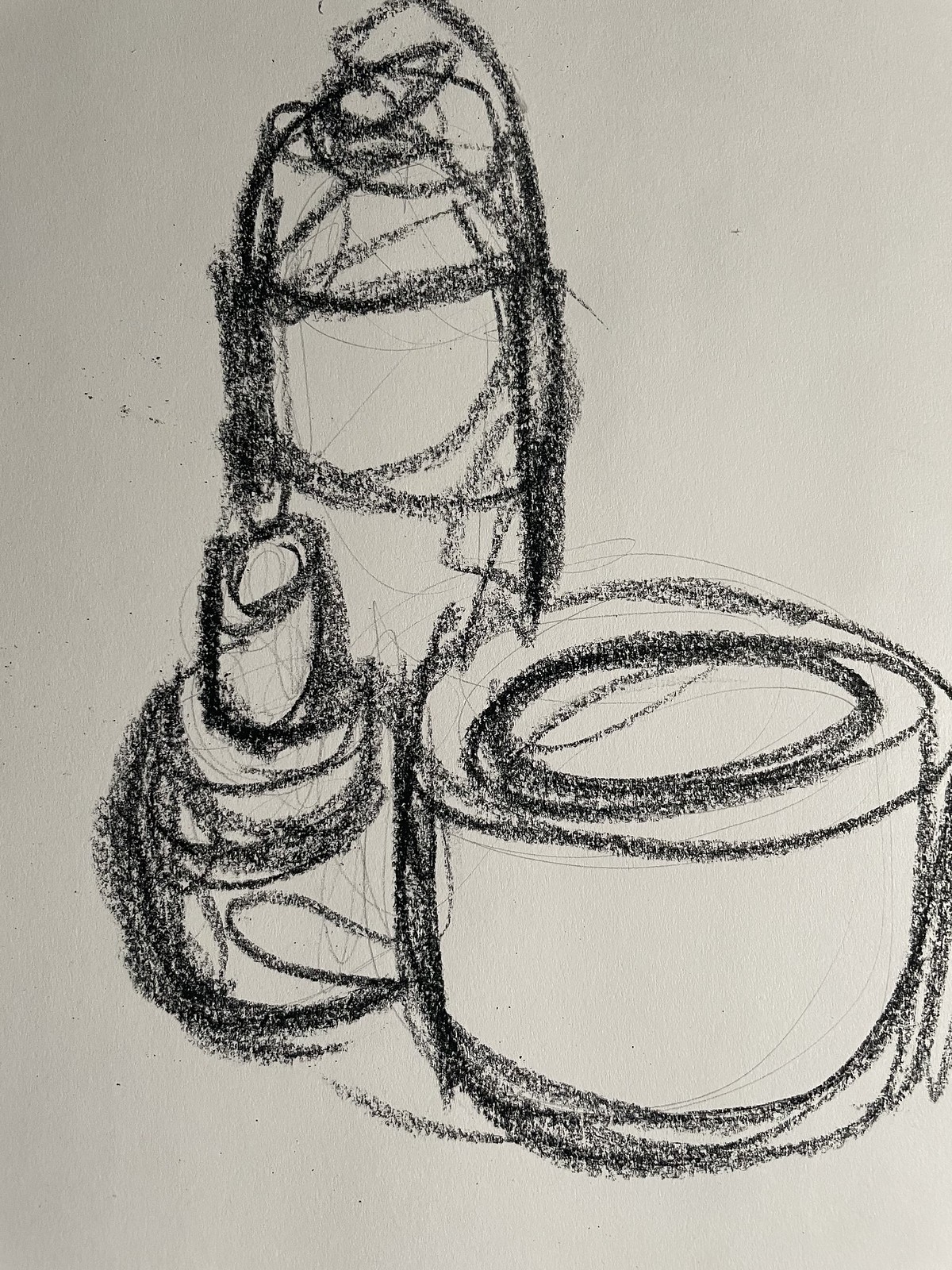The image is a black and white drawing on a piece of construction or drawing paper, likely created with pencil or black crayon. The composition features three distinct objects:

1. In the bottom right corner, there is a cup-shaped object, resembling a bowl or a small cylinder, without any handles or content inside.
2. To the left of this cup, a smaller object is depicted, which looks somewhat similar to a lipstick holder.
3. Positioned centrally behind these two objects is a taller cylindrical form that could be compared to a deodorant container.

The drawing is rudimentary and lacks any text or labels, focusing purely on the shapes and forms of these everyday items.